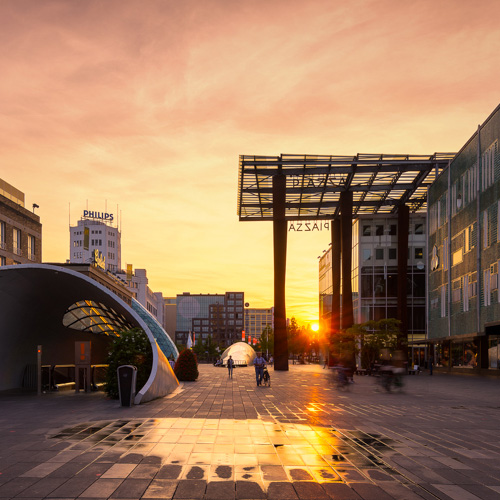This square photograph captures a breathtaking sunset in a bustling plaza in Eindhoven, Netherlands. At the center of the image is a stone-paved plaza with the last rays of the setting sun reflecting off a puddle in the foreground. On the left, a circular structure—likely an entrance to a subway—reveals the top of an escalator descending underground. The plaza is sparsely populated; a few people can be seen walking their dogs and cycling, their motion creating a blur in the image. A prominent canopy, composed of metal bars and supported by six columns, features the word "Piazza" on small signs hanging from either side. Towering in the background is a tall, white skyscraper with the roof-mounted emblem of Philips. The sky transitions beautifully from orange to pink to mauve, capturing the serene yet vibrant end of the day in an urban setting.